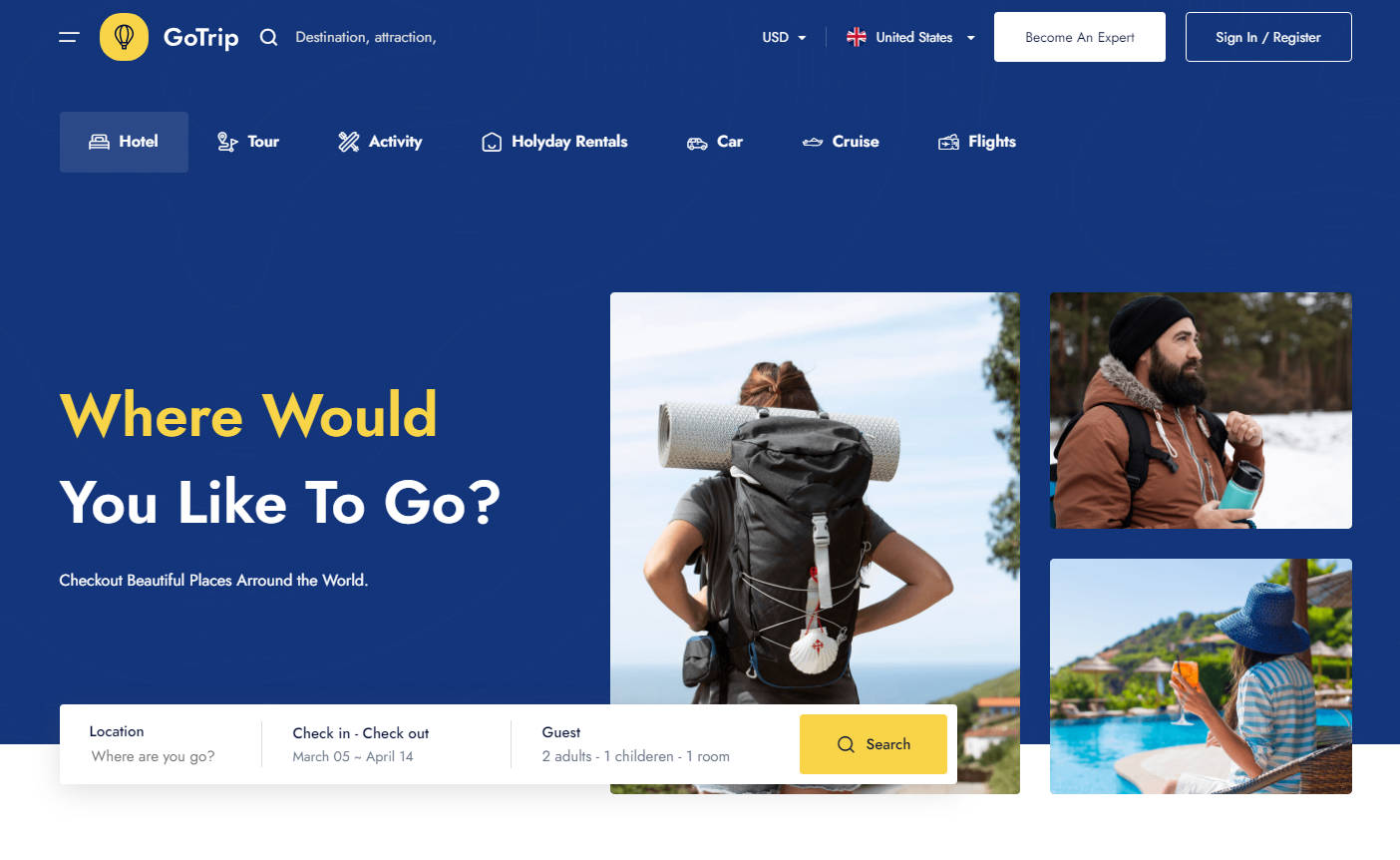The background of the image features a calming blue color, with a prominent yellow circle at the top depicting a hot air balloon. Beside this emblem, the text "Go Trip" is written, accompanied by a search bar area. Below this, there's an interactive white box inscribed with "Become an Expert," and next to it, a blue box offering options to sign in or register.

Beneath these elements, a navigational menu displays words like "Hotel" beside a bed icon, followed by "Tour," "Activity," "Holiday Rentals," "Car," "Cruise," and "Flights." In bold yellow text, the phrase "Where Would?" is written, followed by "You Like to Go?" in white text and the tagline "Check out beautiful places around the world."

At the bottom, there's an interactive section allowing users to enter details for location, check-in and check-out dates, number of guests, and a yellow search bar.

Above this area, a large, expressive image captures a person with a hiking backpack against a backdrop of clouds and distant trees. To the top right, a smaller image shows a bearded man in a black hat and brown jacket, holding a water bottle, set against a snowy landscape with trees. Below this image, a serene scene showcases a woman sitting by a vast swimming pool, wearing a blue hat and holding an orange cup in her hand.